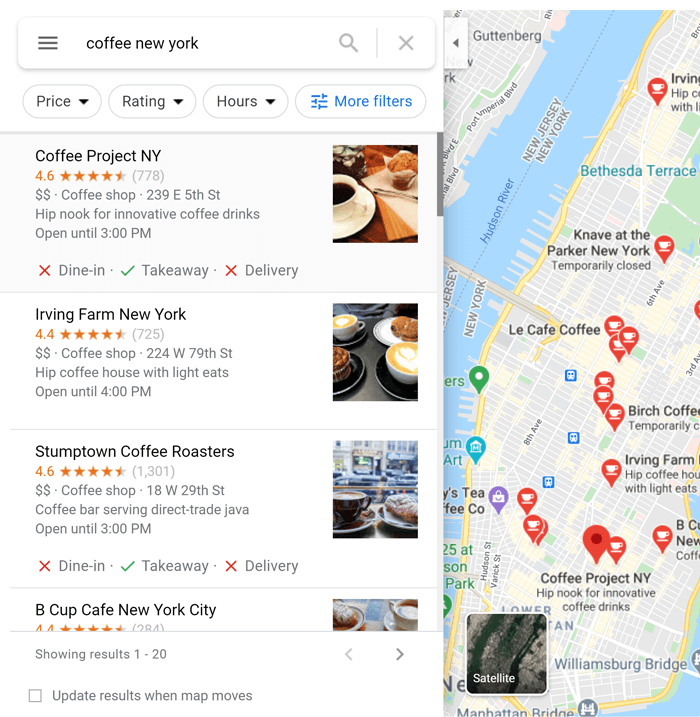This screenshot from Google Maps features a search for coffee shops in New York City, likely in the Lower East Side area, with a portion of Central Park visible. The left side of the screen displays a map dotted with red location markers indicating various coffee shops.

On the left pane, there's a search bar at the top that reads "Coffee New York." Directly below the search bar are four filter tags: Price, Rating, Hours, and More Filters. The search results for coffee shops are listed beneath these filters.

1. **Coffee Project New York**: Located at 239 East 5th Street, this coffee shop has received a rating of 4.6 stars from 778 reviews. It only offers takeout service, with no options for dine-in or delivery.

2. **Irving Farm New York**: This shop, situated at 224 West 79th Street, boasts a 4.4-star rating from 725 reviews. It is open until 4 p.m. and does not offer delivery or dine-in, only takeaway.

3. **Stumptown Coffee Roasters**: With a high rating of 4.6 stars from 1301 reviews, this coffee shop is located at an unspecified address. It provides takeaway service only and is open until 3 p.m.

4. **Bee Cobb Cafe New York City**: Additional details about this shop are not provided in the screenshot.

At the top right corner of the left pane, there's a collapsible tab that allows users to expand or minimize the search results section for "Coffee New York."